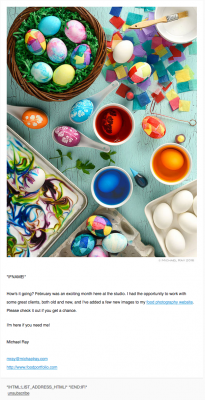This vibrant cell phone screenshot captures a colorful and festive scene centered around Easter egg decorating. Dominating the upper left quadrant, a basket filled with green artificial grass cradles seven pastel and multicolored Easter eggs. Adjacent to the basket in the upper right corner, a scattering of small, colorful squares of paper are partially covered by a white bowl and a paintbrush, suggesting the preparation for crafting.

Moving towards the center, the image showcases three cups filled with vivid red, blue, and yellow dyes, alongside three beautifully decorated eggs in shades of blue, purple, and orange, each adorned with delicate white flower patterns. 

In the bottom left, part of a baking pan is visible, containing a white substance with a chaotic swirl of blue, green, and purple colors indicative of a playful mixing experiment. Below this, three eggs are patterned in a checkered design with various colors, although one remains plain white. 

Finally, occupying the lower right corner, four eggs peek out from a neat compartment within a box. Beneath the image is a small block of text, too tiny to decipher clearly, but it appears to start with a friendly greeting and mentions February being an exciting month for a certain studio, highlighting work with great clients, both old and new. The text ends with a prompt to check out some images and an open offer for further contact, followed by what seems to be a sign-off from "Mother Roy" and two clickable email links.